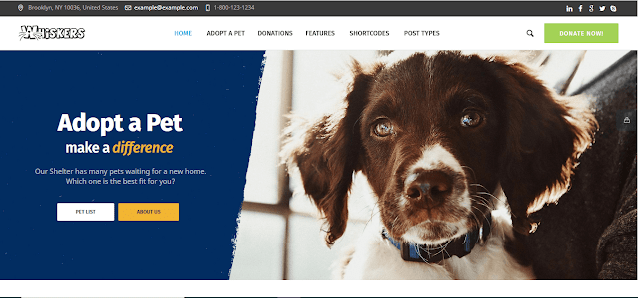This image, sourced from the Whiskers website, features a horizontally rectangular layout. At the top of the site, a thin black banner spans the entire width, displaying essential contact information. On the left side of the banner, a location icon is followed by the text "Brooklyn, New York, 10036 United States," along with a phone number. To the right, social media icons for Whiskers are displayed, including LinkedIn, Facebook, Google, X, and an unrecognizable one.

Beneath the banner, the backdrop switches to a white background. On the left, the website’s name "Whiskers" appears in bold white letters with a navy blue border. Notably, the 'W' in "Whiskers" features cat whiskers extending from its sides. To the right of the title, a horizontal menu offers options: Home, Adopt a Pet, Donations, Features, Shortcodes, and Post Types. Further to the right, a magnifying glass icon allows users to search the site, while a green "Donate Now" button stands out prominently.

The main visual attraction below these menus is a high-resolution image of an adorable dog. This endearing canine looks directly at the camera with soulful brown eyes. It has a predominantly brown face, accented with a touch of white around the nose and a white neck and chest. Its floppy brown ears frame its face, and a blue collar adorns its neck.

Adjacent to the dog, set against a vibrant blue background, the text "Adopt a Pet, Make a Difference" is written in white, with the word "Difference" highlighted in orange. Below, in smaller white text, it reads, "Our shelter has many pets waiting for a new home, which one is the best fit for you?" Two buttons are positioned underneath this text: a white "Pet List" button on the left and an orange "About Us" button on the right.